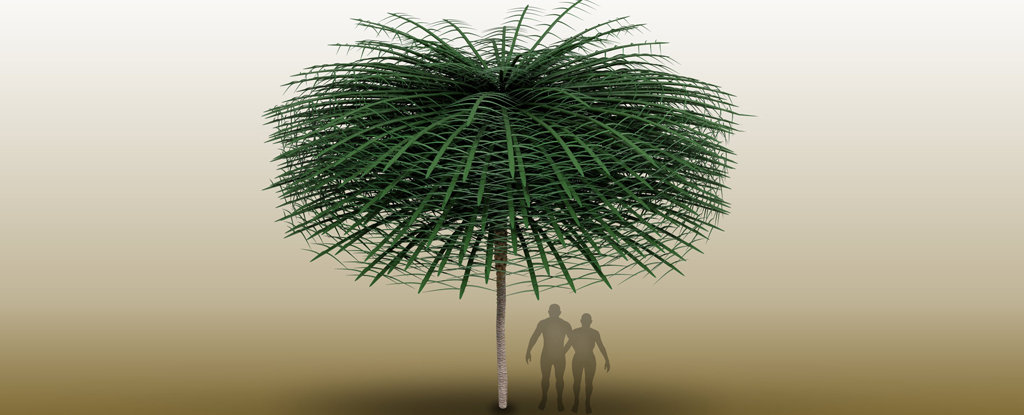The image presents a detailed 3D rendering of a tree centered within a long horizontal frame. The tree, with its thin trunk, extends upwards to display pointy, green branches. These branches resemble palm tree fronds but in a stylized, digital manner, featuring straight green lines with thorny offshoots. Positioned beneath the tree on the right side are two human silhouettes in an A-pose, standing close together. One silhouette is taller and appears male, while the shorter one is possibly female, based on subtle body curves. The figures are stark, bald, and featureless, rendered entirely in dark gray, contrasting sharply against the light gold to tan gradient backdrop. The gradient background transitions from nearly white at the top to a darker tan at the bottom, where a circular shadow under the tree further accentuates the tree's digital design. The overall impression is that of an abstract, computer-generated scene, potentially from a textbook or video screenshot, with minimal yet striking details.